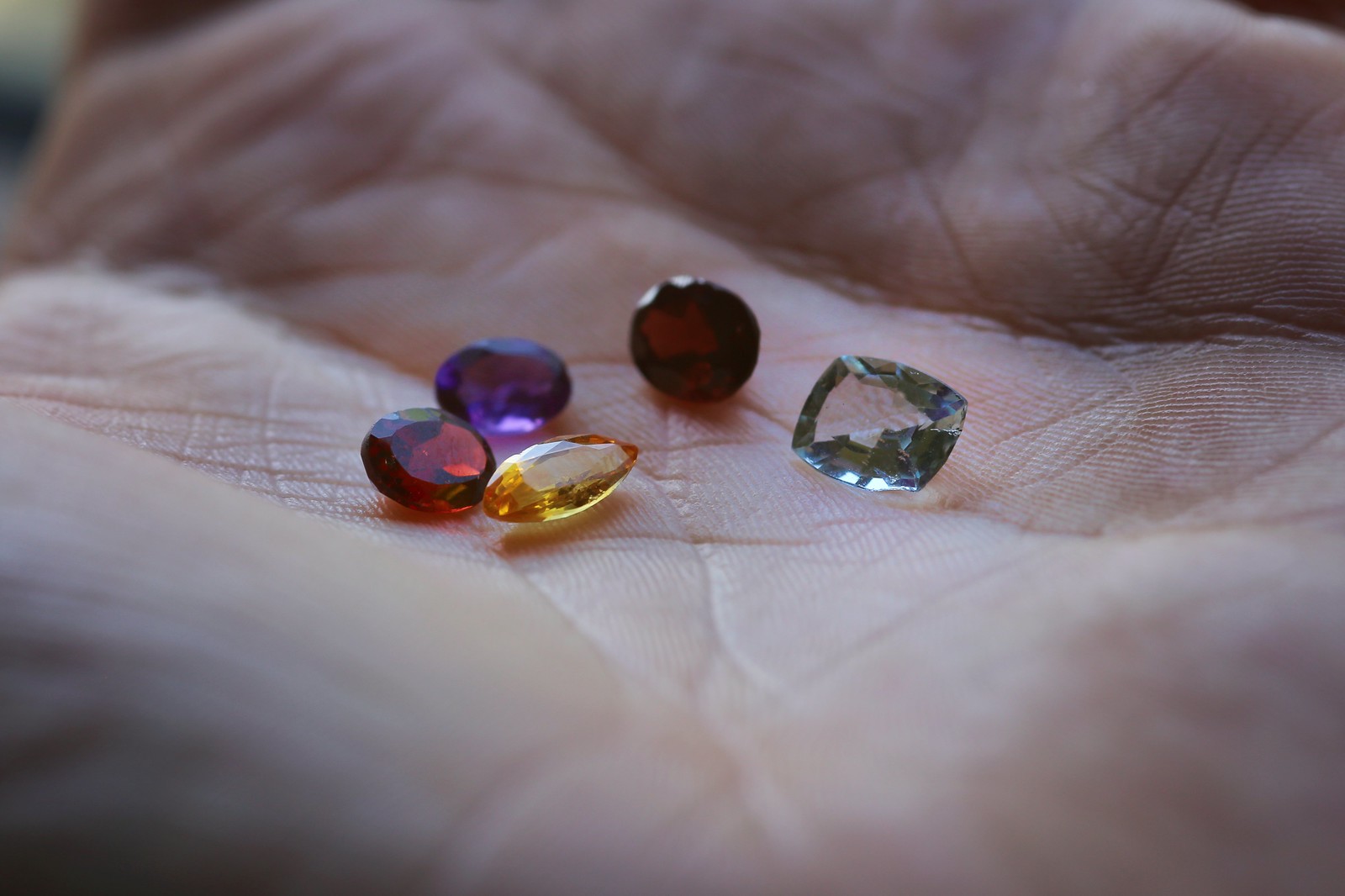This highly detailed, close-up photograph captures five faceted gemstones resting in the palm of an adult's fair-skinned hand, showcased against a blurred teal, blue, and white background. The palm, prominently filling the frame, features numerous visible lines and wrinkles. Among the gems, three are perfectly round - one dark red, potentially a ruby, one ultraviolet purple, and another deep red appearing slightly tilted. Additionally, there is a yellow gem cut into an oval or teardrop shape, and a clear, diamond-like gem with a square shape and subtly curved sides. The intricate details of both the gemstones and the skin's texture are vividly captured, emphasizing the natural contours and hues.